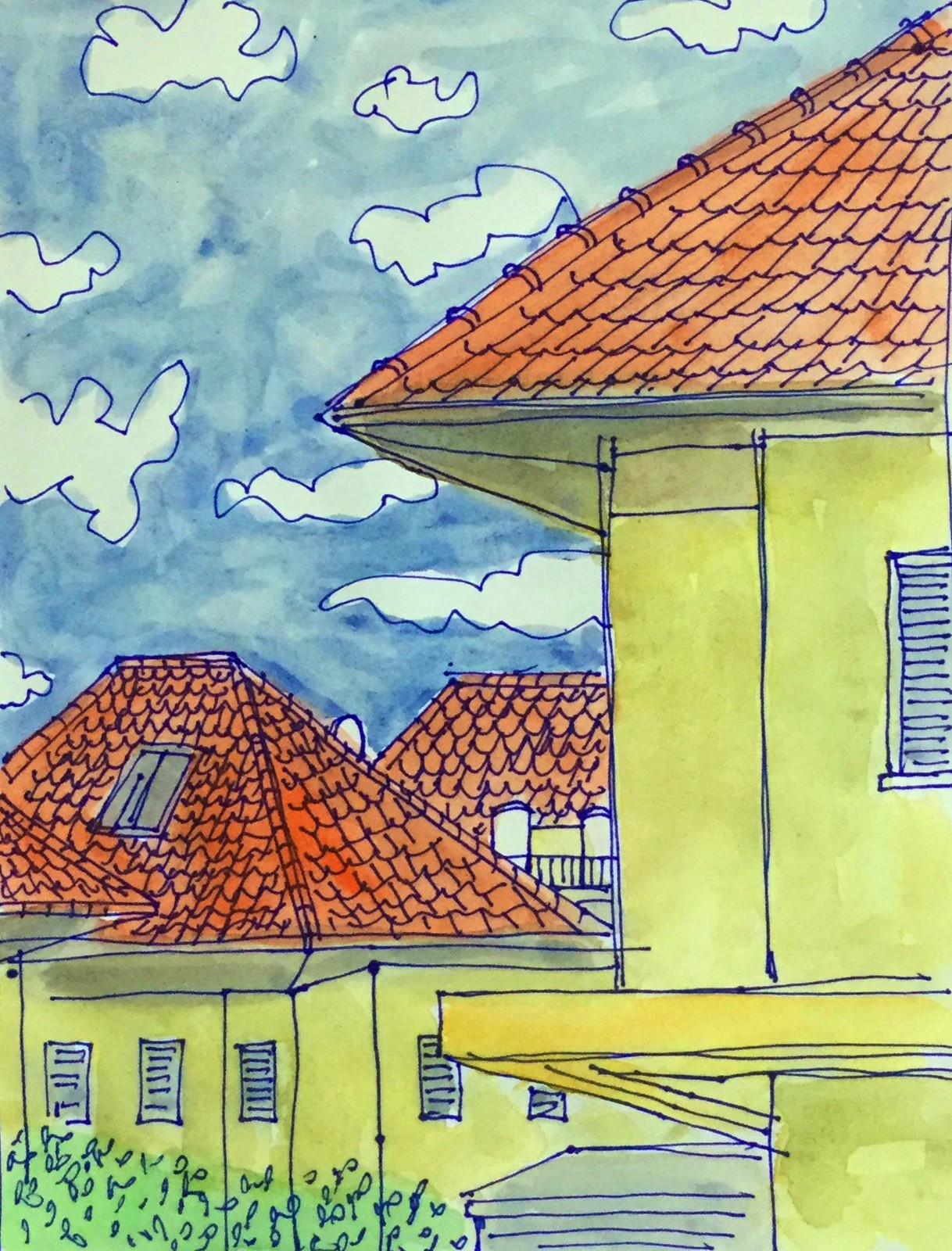This artwork is a vibrant watercolor painting that captures a picturesque scene of clustered buildings or houses. The entire composition is defined by delicate blue ink outlines, creating a cohesive and fluid structure throughout the piece. The sky above is painted in a soft, serene blue, with carefully preserved white spaces mimicking the presence of fluffy clouds drifting across the horizon. Numerous buildings grace the painting, predominantly in warm, inviting shades of yellow. Among them is a prominent two-story structure, drawing the viewer's eye with its height and prominence. The roofs of these charming houses are adorned with a rusty orange hue, suggestive of terracotta tiles, adding a touch of rustic elegance to the scene. At the ground level, lush green grass and verdant plants infuse the painting with life and natural beauty, grounding the architectural elements in a serene, almost idyllic setting.